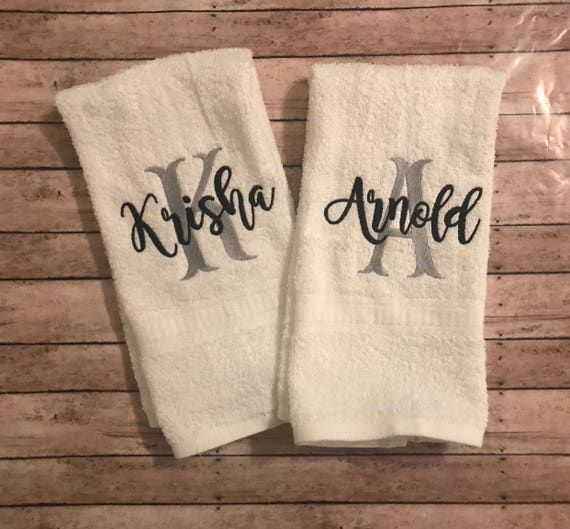This image showcases a set of two monogrammed hand towels, elegantly displayed against a backdrop of wooden slats with visible grain lines. Both towels are a light beige color, adding a touch of subtle sophistication. The towel on the left features a large grey capital "K" with the name "Krisha" intricately embroidered in black cursive script across it, spelling K-R-I-S-H-A. Similarly, the towel on the right displays a large grey capital "A" with the name "Arnold" embroidered in the same black cursive, spelling A-R-N-O-L-D. The ambient light, possibly reflecting from the ceiling, adds a gentle highlight to the scene, enhancing the texture of the wooden surface.